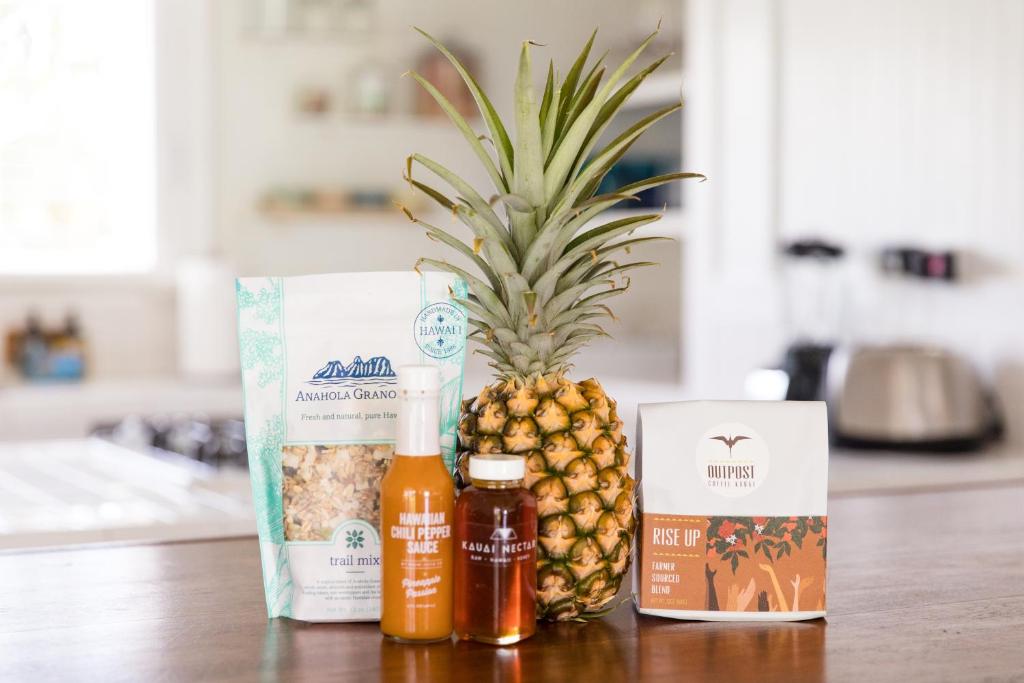This close-up product shot showcases a vibrant scene on a wooden kitchen counter, featuring a central pineapple flanked by two distinct bags of granola. The granola packages include a taller, white bag labeled Anahola Granola with a blue and teal design, and another white bag branded Outpost Rise Up, adorned with illustrations of hands reaching up to a floral tree. In the foreground, in front of the pineapple, sit two small glass jars: one containing golden honey, labeled Kauai Nectar, with a white lid, and the other holding an unopened, orange Hawaiian chili pepper sauce. The background, softly blurred, reveals kitchen shelves and a stove, with sunlight streaming through a window on the left, where a roll of paper towels sits on the counter. This rich tableau evokes a sense of Hawaiian culinary tradition and homey comfort.